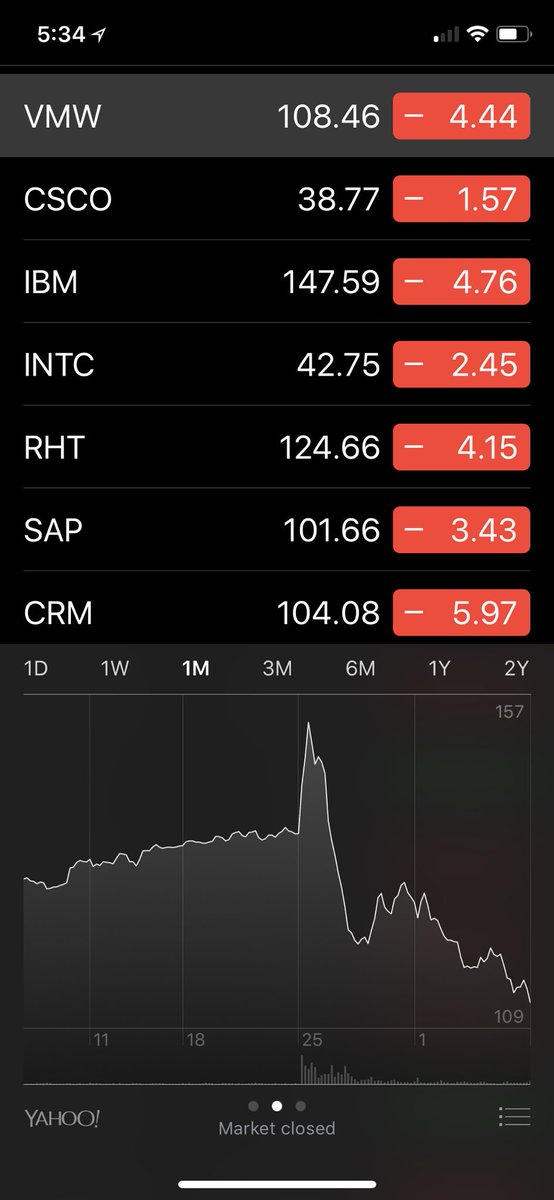The image showcases a tablet or cell phone displaying a stock market tracking application on a predominantly black background. At the top of the screen, in white text, it displays the time as "5:34." The status bar indicates a network signal strength of 1 out of 4 bars, full Wi-Fi connectivity, and a battery level just above half. 

The stock information starts with VMW, whose current price is $108.46, marked by a drop of -4.44. This decrease is highlighted in a red rectangle, and the VMW stock is also highlighted in a light gray color, distinct from the others. The following stocks are listed on a black background, each showing a downward trend with the decreases also indicated within red rectangles:

- CSCO: $38.77, down -1.57
- IBM: $147.59, down -4.76
- INTC: $42.75, down -2.45
- RHT: $124.66, down -4.15
- SAP: $101.66, down -3.43
- CRM: $104.08, down -5.97

Below the list of stocks, there is a line graph representing the market trends. At the bottom of the screen, it states "Yahoo" and "market closed," indicating the source of the information and the current market status.